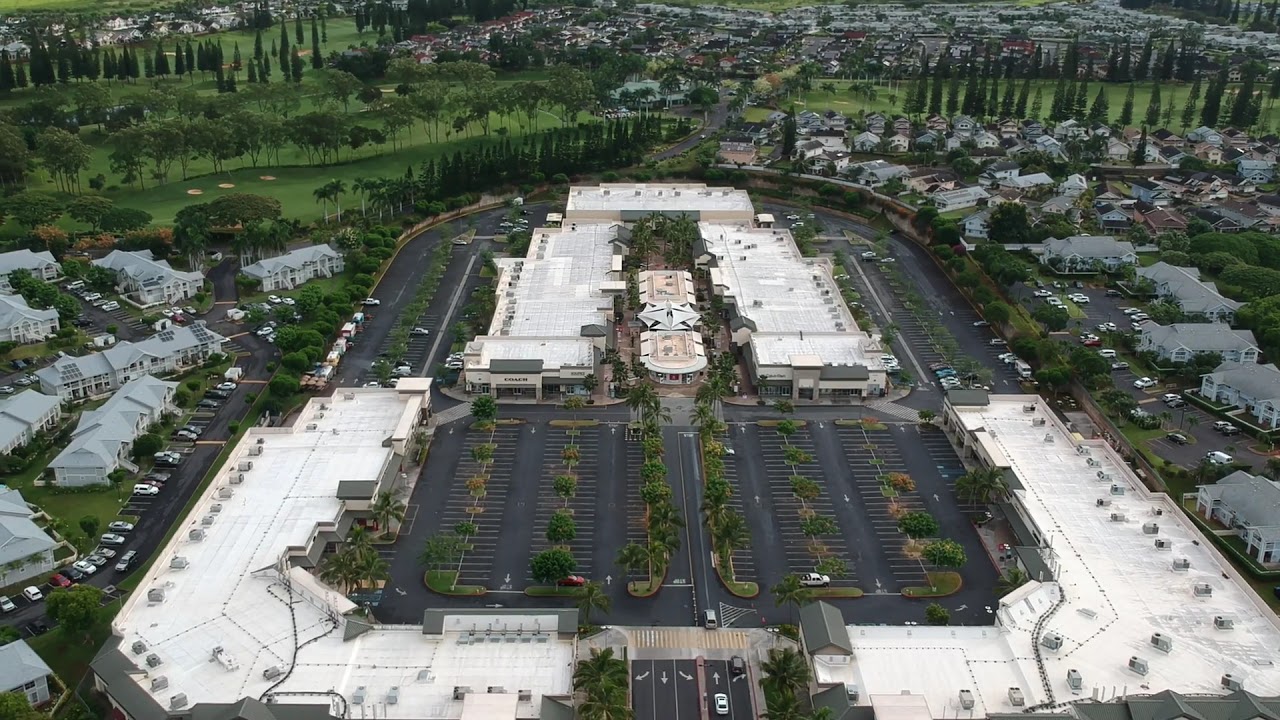This aerial view, possibly captured by a drone, showcases a large, upscale outdoor shopping mall nestled within a residential neighborhood. The mall complex forms an almost U-shaped arrangement of interconnected buildings, with a vast central courtyard and parking lots lined with manicured palm trees, contributing to its refined ambiance. Surrounding the mall, there's an abundance of residential homes with red tile roofs, closely packed together, indicative of a high-end community. The scene also includes a prominent golf course in the background, featuring meticulously planted trees, Italian cypress, sand traps, and a central pond, further enhancing the area’s upscale aesthetic. The mall is flanked by additional office buildings and offers extensive parking areas, reinforcing its accessibility and convenience within this lavish setting.